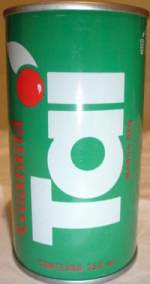This tightly cropped photograph features a vibrant green can, prominently showcasing the bold, white block letters "T-A-L" across its midsection. The can is bordered at the top and bottom with silver linings, adding a metallic contrast to its overall appearance. Above the letter 'L,' there is a distinctive red circle accompanied by a white protrusion resembling a leaf. The background, barely visible, hints at a wooden texture in a brown hue. Additional text appears on both the lower left and right of the can, but it remains indecipherable due to significant blurriness. The design element on the left side of the can is notably larger compared to the right.